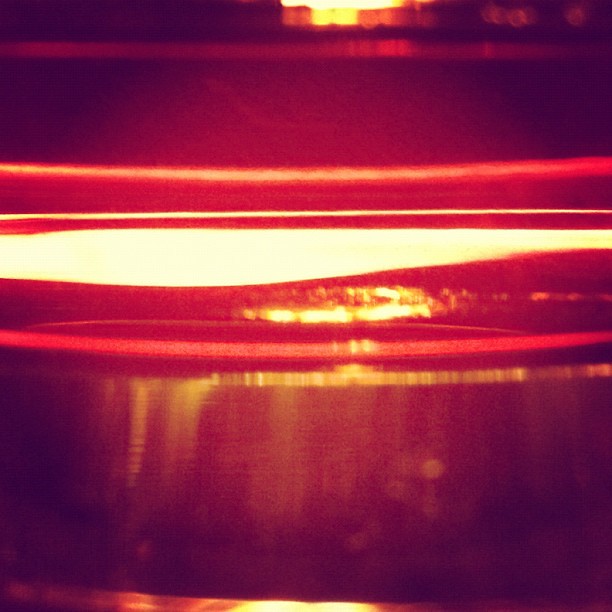This image evokes a sense of ambiguity, marked by a blend of glowing colors and abstract shapes. Dominating the scene is a vibrant disc-shaped glow of yellow and red, reminiscent of a nuclear explosion's iconic mushroom cloud, yet clearly something else upon closer inspection. This glowing form sits above a dark, rounded structure that could be interpreted as a large metal plate or possibly the surface of water. The intense heat-like distortion adds to the enigmatic quality of the image.

A prominent yellow streak cuts horizontally across the center, widening towards the left, further adding to the surreal effect. At the top of the image, a yellow light appears to shine downward, casting an eerie glow over the scene. The overall palette transitions from deep reds and maroons at the top, through the central bright glow, to a darker, red-tinged lower half, creating a gradient effect that is both warm and intense.

In summary, the image is a complex tapestry of glowing yellows, reds, and maroons with a central luminous streak, presenting a scene that's open to interpretation, whether seen as a heated glass distortion, a fiery landscape, or a surreal sunset over a dark, reflective surface.